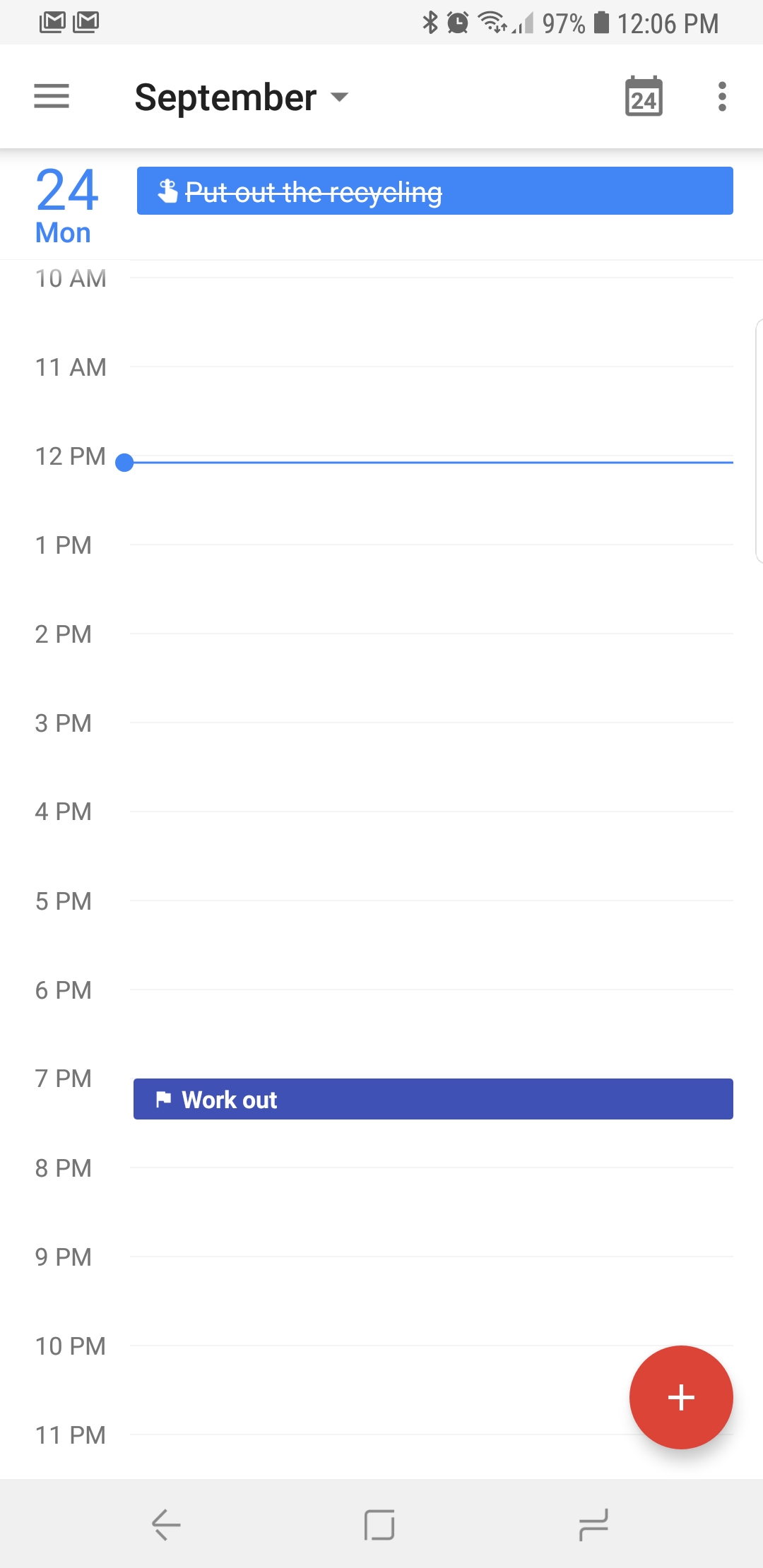The image depicts a screenshot from a smartphone, characterized by a tall, narrow rectangular shape. At the top of the screen, the date is displayed in large font, indicating "September 24th," specifically noting that it is a Monday. Accompanying the date are common smartphone icons, including battery life and the time, which reads 12:06 PM.

Further down, next to the date, a text reminder states "Put out the recycling," accompanied by a pointing finger icon. This task has been crossed out, signifying its completion. 

The screen also features a detailed hourly schedule beginning at 10 AM and continuing through to 11 PM, listed in sequential order. Notably, at 7 PM, there's a task labeled "Work out." At the bottom of the screen, a red plus sign is visible, likely indicating an option to add more tasks or events.